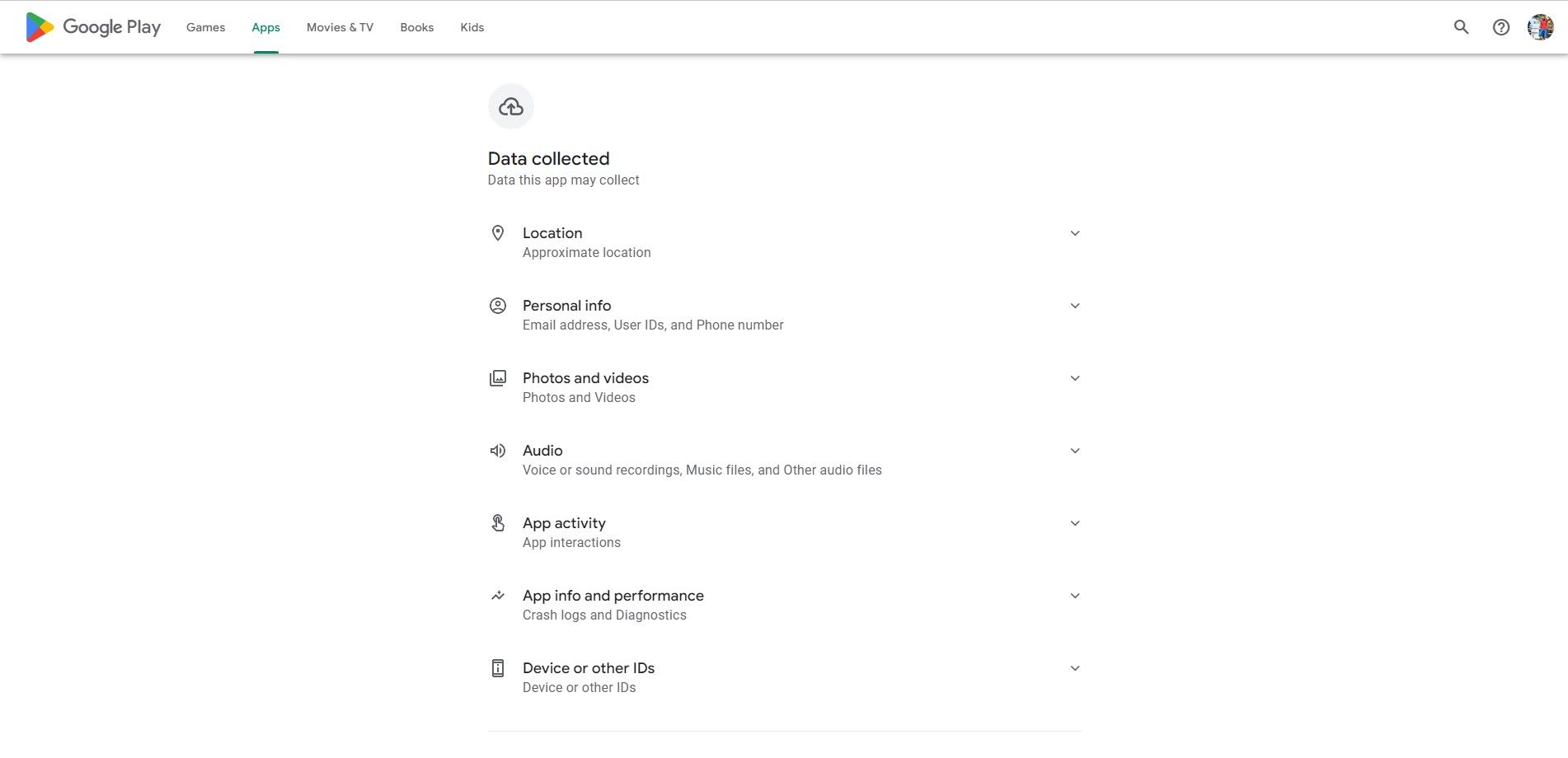A screen capture of the Google Play interface on a white background. At the top is the Google Play logo featuring a play button in shades of pink, gold, and teal. Below the logo, navigation options are visible: Games, Apps, Movies & TV, Books, and Kids, accompanied by icons for a magnifying glass, a question mark in a circle, and a profile picture that is too small to discern clearly. 

Centrally aligned text in gray indicates "Data collected," followed by "Data this app may collect," with dropdown arrows next to each heading. The first category, "Location," has an icon of a location pin and notes "Approximate location." Next, "Personal info" is denoted by a person icon and includes "Email address," "User IDs," and "Phone number." "Photos and videos" follow, marked by a square icon and labeled "Photos and videos."

The "Audio" category includes a speaker icon and lists "Voice or sound recordings," "Music files," and "Other audio files." "App activity," illustrated with an icon that resembles a duck, notes "App interactions." "App info and performance," showing a wave-like icon, mentions "Crash logs and diagnostics." The final category, "Device or other IDs," is marked with a cell phone icon and labeled "Device or other IDs."